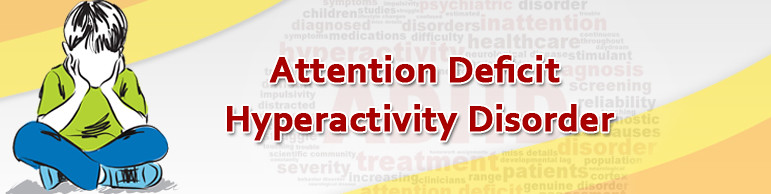The image is a long rectangular informational banner featuring an illustrated cartoon of a boy sitting cross-legged on the ground. The boy has short black hair and no facial features, and he is drawn in black and wears a bright green shirt, blue jeans, and light blue sneakers. He is resting his chin in his hands and appears to look bored or pensive. The banner has a gradient background with a small orange triangle in the upper left corner, followed by a yellow ribbon beneath it, gradually transitioning back to yellow and orange on the right side. 

The middle of the banner is predominantly white and contains a prominent red text with a white border stating "Attention Deficit Hyperactivity Disorder." Behind this main text is a semi-transparent word cloud in red and black, with various words related to mental health and ADHD, such as "diagnosed," "inattention," "healthcare," "disorder," "psychiatric disorders," "treatment," "patients," and more. The overall design and elements emphasize the theme of ADHD and its related concepts.